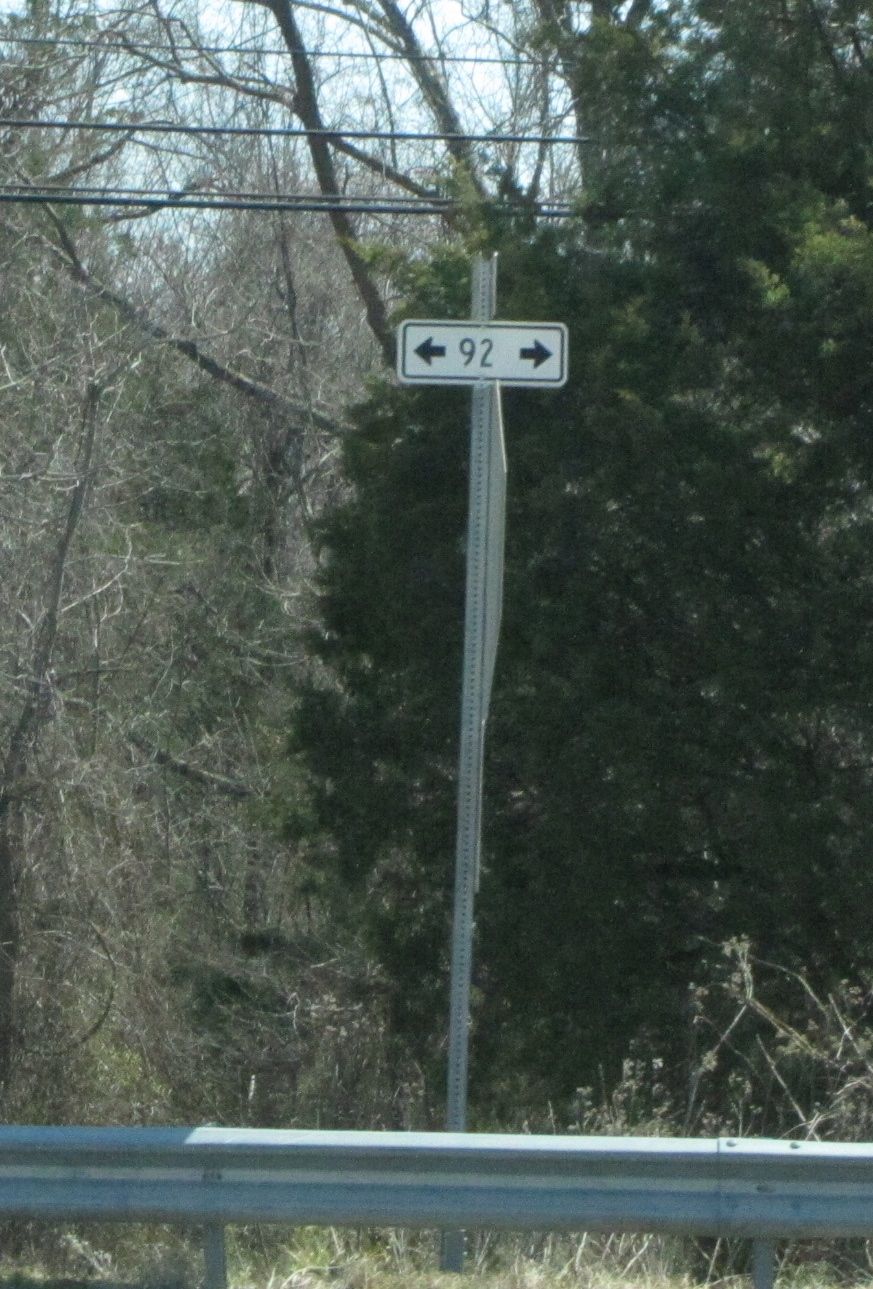This digital photograph, taken from a roadway, depicts a scene dominated by contrasting elements of nature and infrastructure. At the bottom of the image, a thick silver guardrail lines the road, providing a clear boundary. Beyond the guardrail, various trees create a stark visual dichotomy; while the trees on the left side of the frame are bare, revealing their brown branches and trunks, the trees on the right are lush and green, including a prominent pine tree. Tall, tan weeds also occupy the foreground, enhancing the natural aspects of the scene.

A silver pole rises from the grass at the bottom and holds a small, rectangular white sign marked with the number 92. This central sign features a left-facing arrow before the "9" and a right-facing arrow after the "2", providing directional guidance. Additionally, the upper portion of the photo reveals three power lines stretching across a cloudy, whitish sky, further blending elements of man-made and natural settings. On the right-hand side of the image, the lower half of a hexagonal stop sign is faintly visible behind some vegetation, adding to the intricate details of this roadway scene.